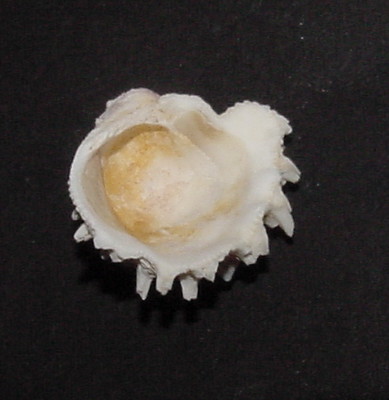This photograph features an off-white seashell displayed on a black fabric background. The seashell has a vaguely heart-like shape with prominent ridges around its sides and spiky, jagged features extending from its edges. Notably, the shell's color transitions from white on the exterior to a more yellowish or golden-brown hue towards the center, suggesting either natural variation or possible dirt accumulation. The seashell's open part is positioned at the forefront, revealing a smooth, slightly swirling interior. There's also an indentation on the left side of the shell. The overall presentation highlights the shell's delicate and sharp features, indicating care must be taken when handling.